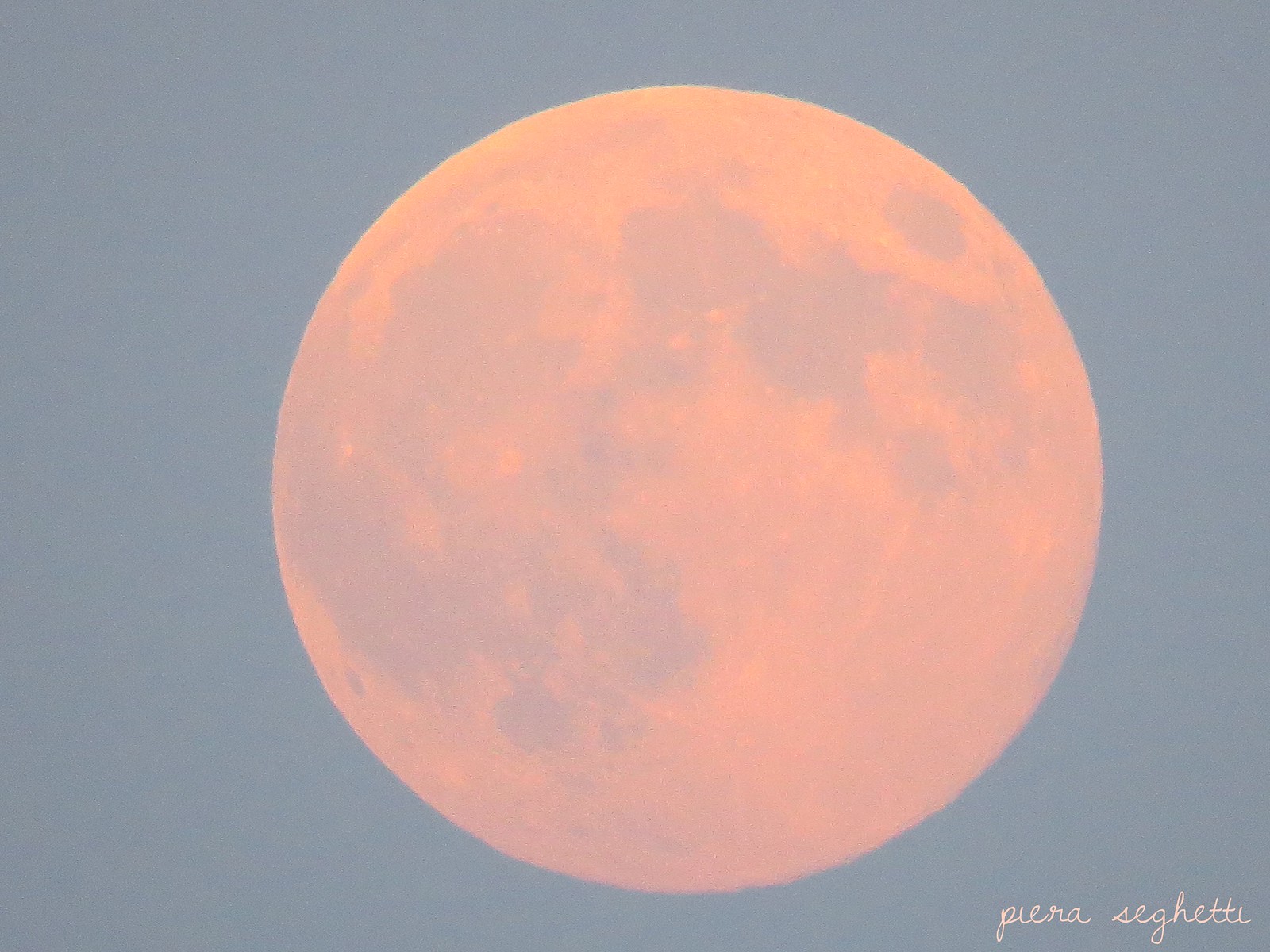This image depicts a large, circular moon centrally positioned against a clear, dark bluish-gray sky that hints at either dawn or dusk. The moon, rendered in a striking light pink-orange hue, is meticulously detailed, showcasing an array of darker splotches that delineate the lunar seas and elevations. The photo's high clarity accentuates these intricate features. At the bottom right, a pink cursive signature—"Piera Seghetti"—graces the image, adding a personal touch from the artist. Though the moon dominates the scene, the overall minimalistic composition, free from clouds or additional celestial bodies, hints at the artistic nature of this well-crafted piece, blurring the lines between a photograph and a potential album cover or painting.